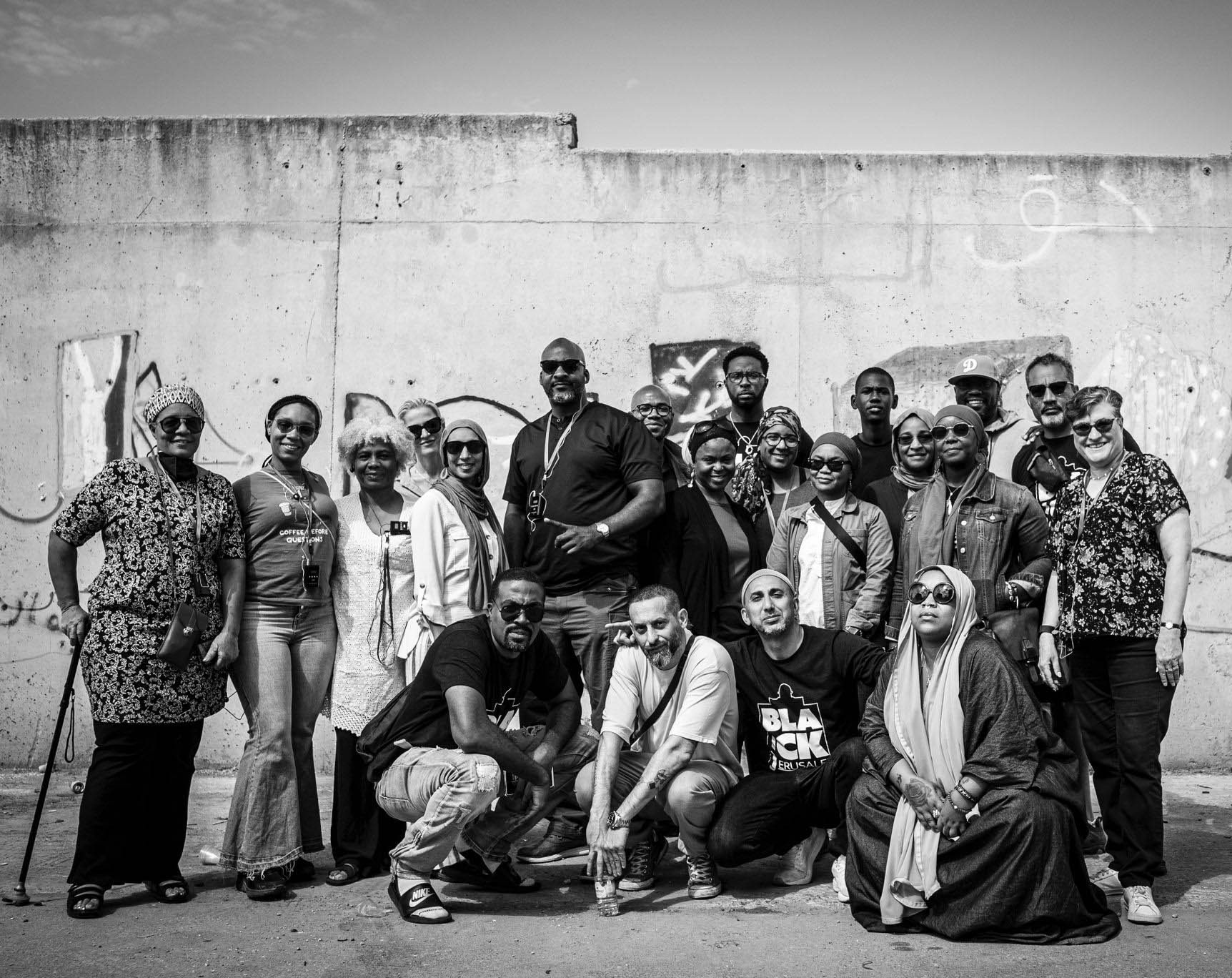This high-quality black-and-white photograph captures a diverse group of around 15 to 20 individuals posing in front of a graffiti-covered block wall. The composition features people from various cultural backgrounds, including African American and Caucasian descent. The group is arranged in two layers: a front row where individuals are either kneeling or sitting, and a back row of standing individuals. Among the women, several are wearing head coverings such as hijabs, while some men are distinguished by their clothing, including a tall African American man in a black shirt. One notable feature is a man with a shirt bearing the word "black." The image showcases different styles among the group, with floral patterns and both lighter and darker skin tones visible. The wall behind them is aged and marked by different shades of darkness and distinct white and black graffiti, further adding to the image's gritty atmosphere. A light sky with faint clouds occupies the top left of the frame. The people’s varied expressions and poses, such as the front man in white with a defiant stance and a woman holding a cane, add to the rich tapestry of this seemingly candid yet purposeful gathering in what appears to be an urban setting marked by the distressed cement wall and roadway beneath them.